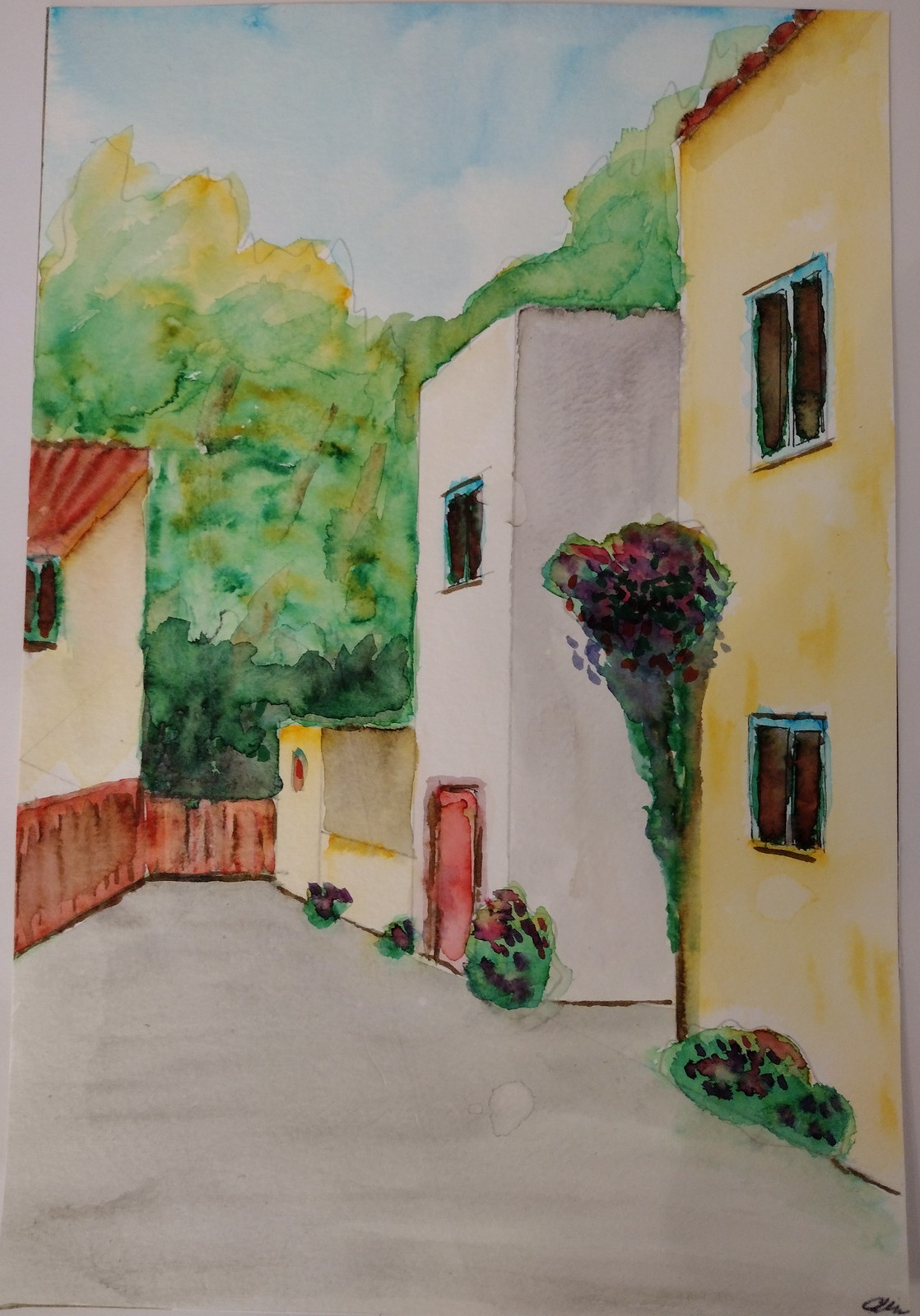The drawing illustrates a quaint urban alley lined with trees in the background. The walkway appears to be pedestrian-friendly, rather than accessible to vehicles. On the right side, there are two two-story buildings; the furthest one is white with a blue-framed window on the upper floor and an entry door in an off-red, orange hue below. Adjacent to it is a single-story structure that seems like a patio wall. The nearest building on the right features windows on both floors, is painted in a mix of off-burnt yellow and white, and does not have a visible door. On the left side, a one-story building, possibly the back of a trailer, is partially visible, displaying only a window. The scene is adorned with shrubs and a tall flowering plant in front of the buildings on the right, nearly reaching the second-story window sill.